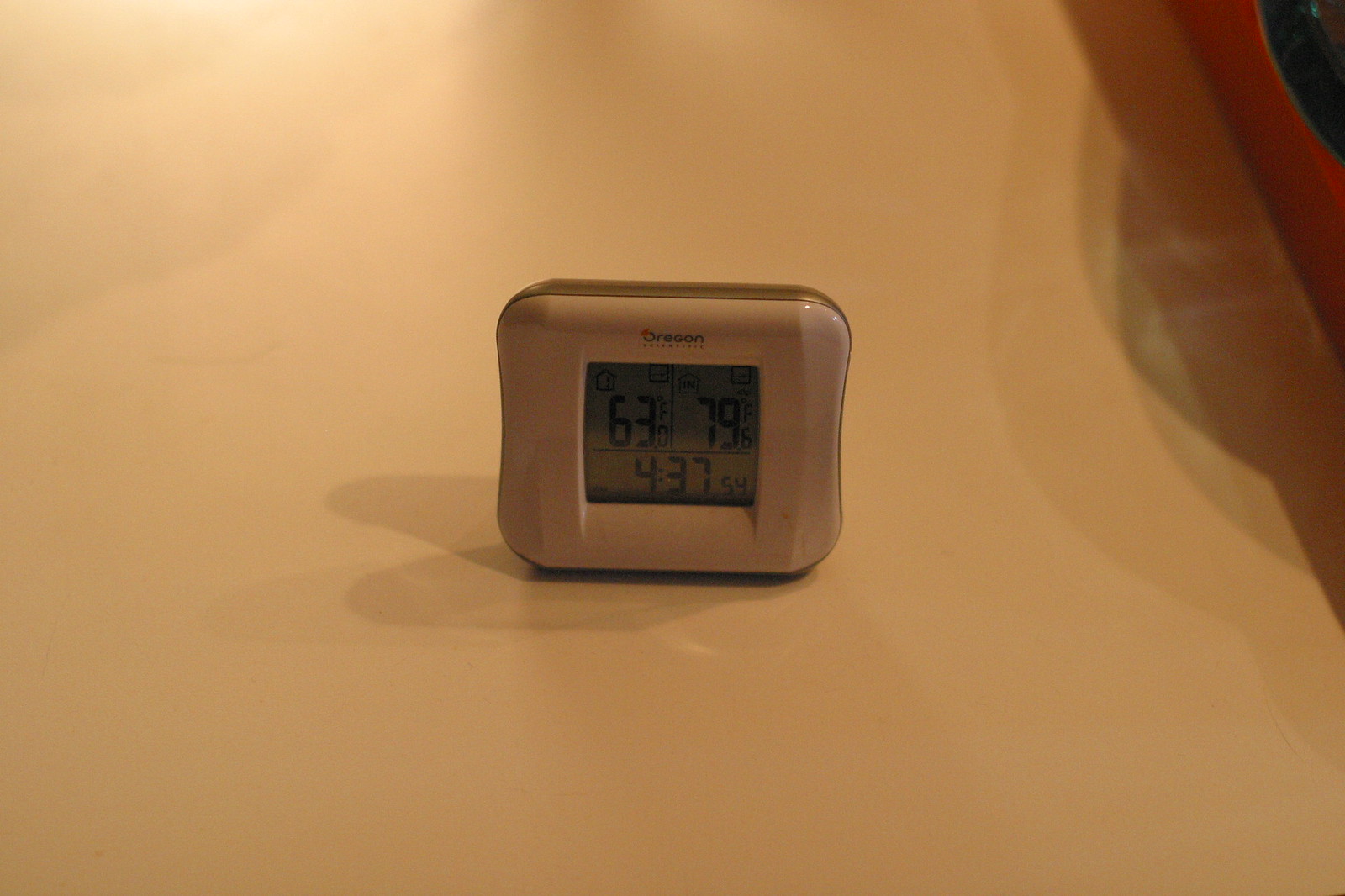A detailed description of the image depicts a white surface, possibly the interior of a box or the top of a table, with noticeable shadowing on the right side suggesting an adjacent edge. Dominating the center of the scene is a small plastic device, resembling a digital thermostat typically wall-mounted but currently positioned vertically on the flat surface, as indicated by the shadow behind it. The device's display shows various information: on the upper left, there is a house icon accompanied by "63F" and the letter "O", while on the upper right, another house icon is displayed along with "79F6". Additionally, the bottom section of the device features a time reading, "4...3754". This suggests that the device likely monitors or controls temperature, providing readings for different zones within a house.